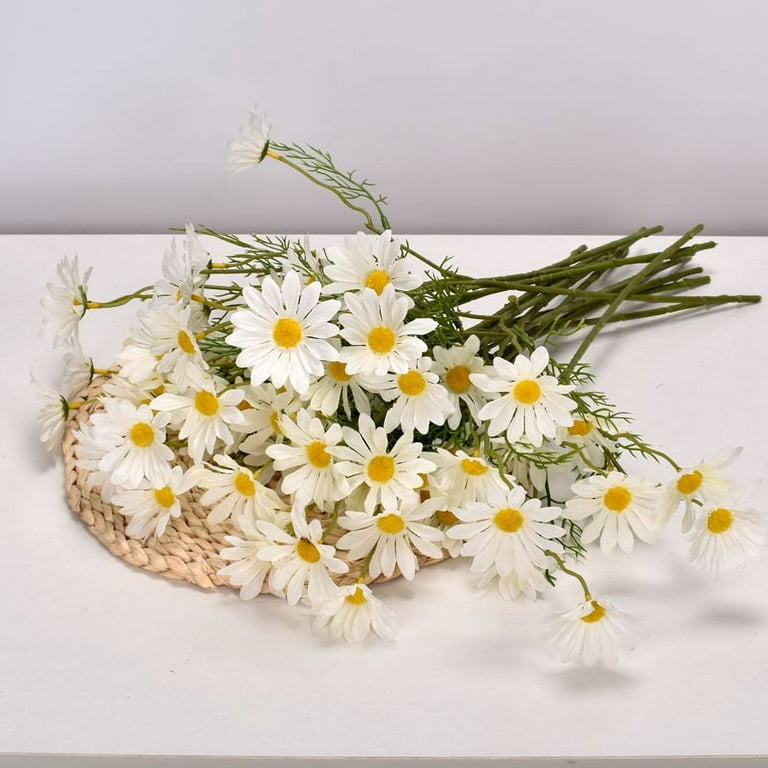In a minimalist studio setup, a bouquet of daffodils is artfully arranged against a pristine white backdrop, consisting of both a white wall and a white floor. The flowers themselves appear fresh and healthy, exhibiting no signs of wilting. The daffodils feature vibrant white petals with sunny yellow centers, complemented by slender green stems and delicate green offshoots. The bouquet seems to have been casually placed or perhaps dropped onto a rustic straw hat or straw placemat, which serves as a natural and earthy base for the arrangement. The straw, with its characteristic yellowish hue, contrasts beautifully with the flowers. Some of the daffodils cascade over the straw, creating a sense of movement, while others rest directly on it. On both the left and right sides, a few flowers extend outward or upward, enhancing the informal, freeform nature of the composition, as if captured in a moment of serendipitous beauty.